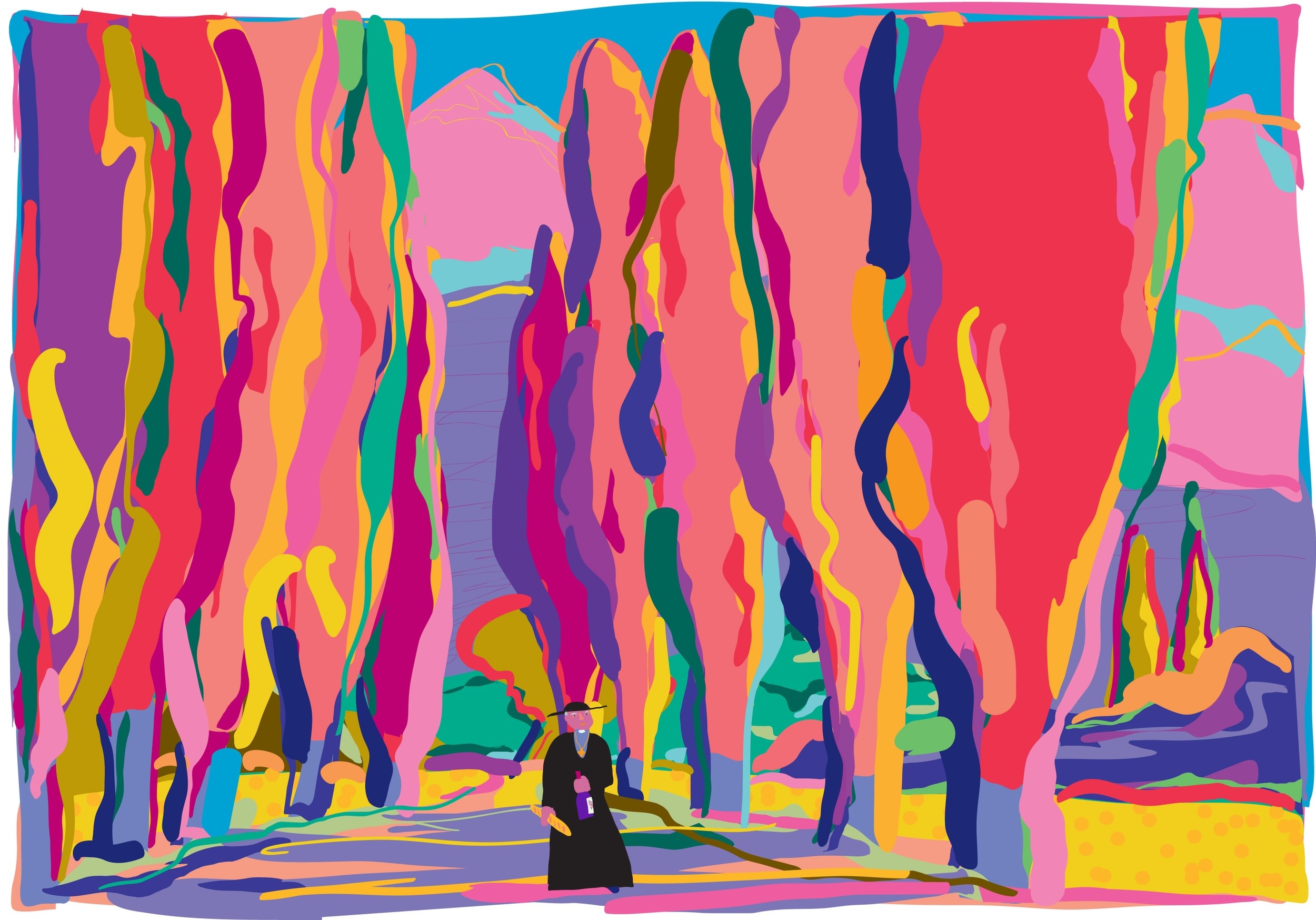This image appears to be a vibrant, abstract painting, characterized by its extensive use of vivid colors. The scene depicts a small figure, likely an ancient Asian man, dressed in black clerical robes and a wide-brimmed black hat, walking down a pathway. He has a long beard and is carrying an oblong yellow object, possibly a loaf of bread, in his right hand, and a bottle, potentially of wine, in his left. The path is flanked by five trees on each side, their broad trunks leading to a cascade of bright, multicolored foliage including hues of red, blue, green, yellow, purple, pink, and peach. These trees appear almost flame-like in their vibrancy. Dominating the left side of the image, these trees create a striking contrast with the purplish mountain and blue sky visible in the background, cementing the painting’s abstract and surreal ambiance.